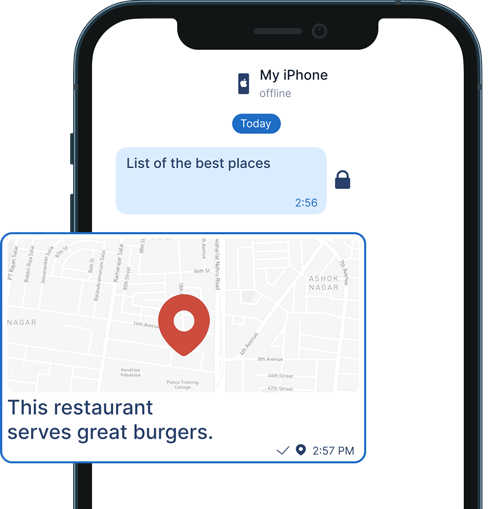The image depicts a smartphone with a black frame. At the top of the phone, there is a black bar, a typical feature of most smartphones. In the center of the screen, the text "My iPhone" is displayed. To the left of these words, the small Apple logo can be seen. Below this, there is a blue box containing the text "Today," and underneath it, another blue box that reads "List of the best places," with the number 256 in the lower right corner of the box. To the right of this number, there is a small lock icon.

Further down, the screen shows a map that appears to be either from Google Maps or Apple Maps. The map displays streets, with "Nagar" being the only street name clearly visible. A prominent red pin is located in the middle of the map, which is outlined in blue. Below the map, in blue letters, it states "This restaurant serves great burgers." In the bottom right corner, there is a checkmark next to the time "2:57 p.m."